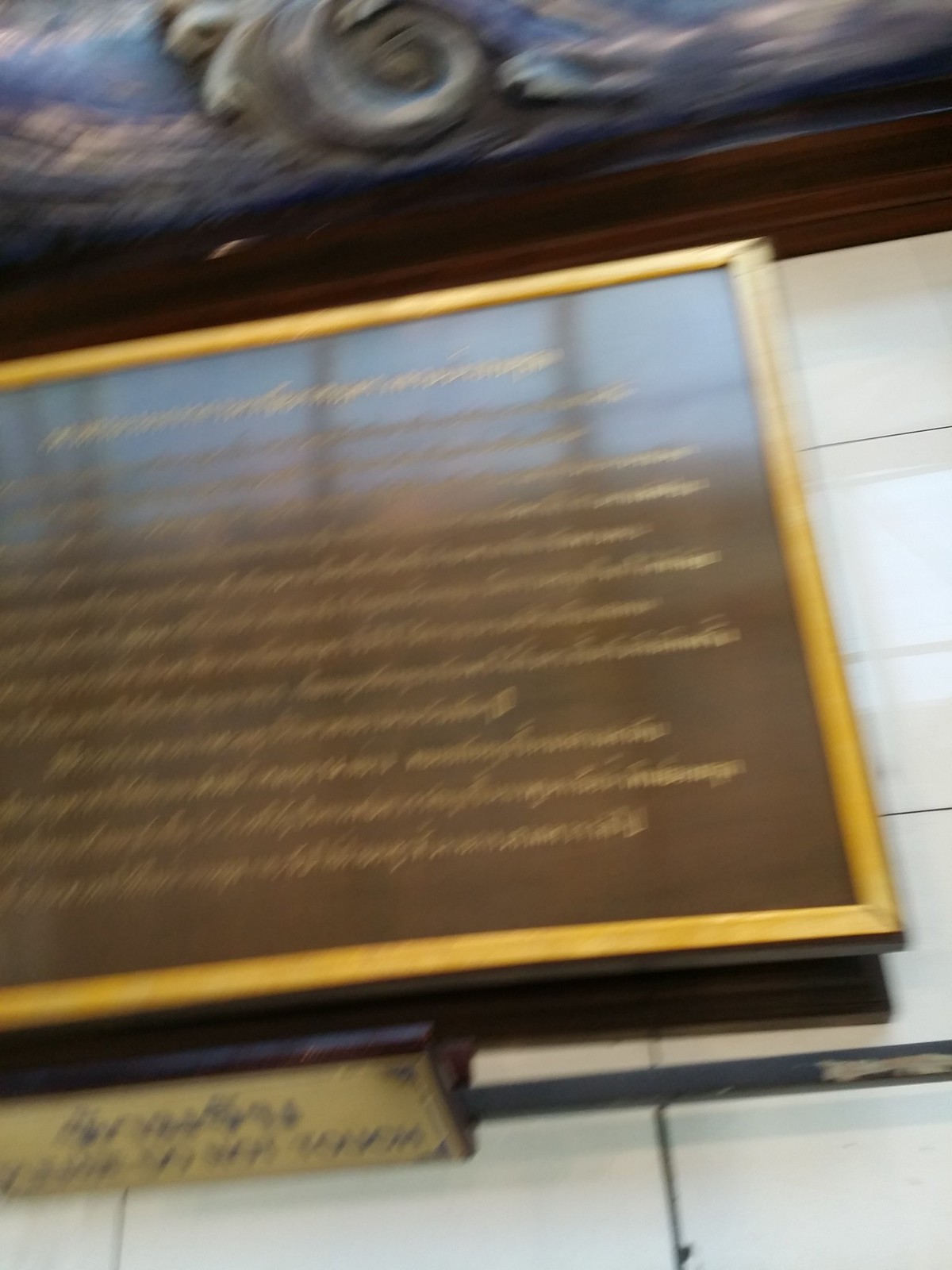This is a close-up, portrait-oriented photograph of a large sign, likely located in a museum. The image appears blurry but several details can be discerned. The sign features a gold border with a brown background and gold cursive lettering, though the blur obscures the exact text. The sign is mounted against a white wall and has a smaller sign positioned directly below it. Above the sign, part of the ceiling is visible, adorned with a blue and gray painting.